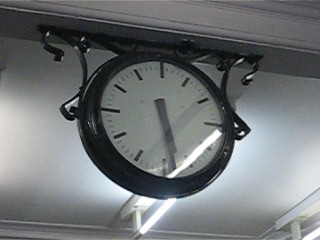This black and white photograph features a meticulously detailed depiction of a hanging clock mounted on a wooden beam. The wooden grain of the beam, despite the monochromatic palette, is discernible, adding a rustic charm to the composition. Centered at the bottom of this beam is the clock, secured in place by a distinct arrangement of metalwork. A rectangular piece of black metal is firmly attached to the beam, and from it emerge elegantly curved metal supports that gracefully descend to cradle the clock.

The clock itself boasts a contrasting design with its black outer casing and stark white face, drawing the viewer's attention. Instead of traditional numbers, the clock face features minimalist hour indicators in the form of lines, with extended markers denoting the 12, 3, 6, and 9 o'clock positions. The slender black hands stand out sharply against the white backdrop, ensuring easy readability.

Adding a touch of industrial modernity, to the right and slightly below the clock, a fluorescent light bulb stretches horizontally across the ceiling, intersecting the otherwise rustic and classical elements of the photograph. The juxtaposition of the wooden beam, vintage clock design, and modern fluorescent light creates a captivating visual narrative, blending differing eras and styles in a single frame.